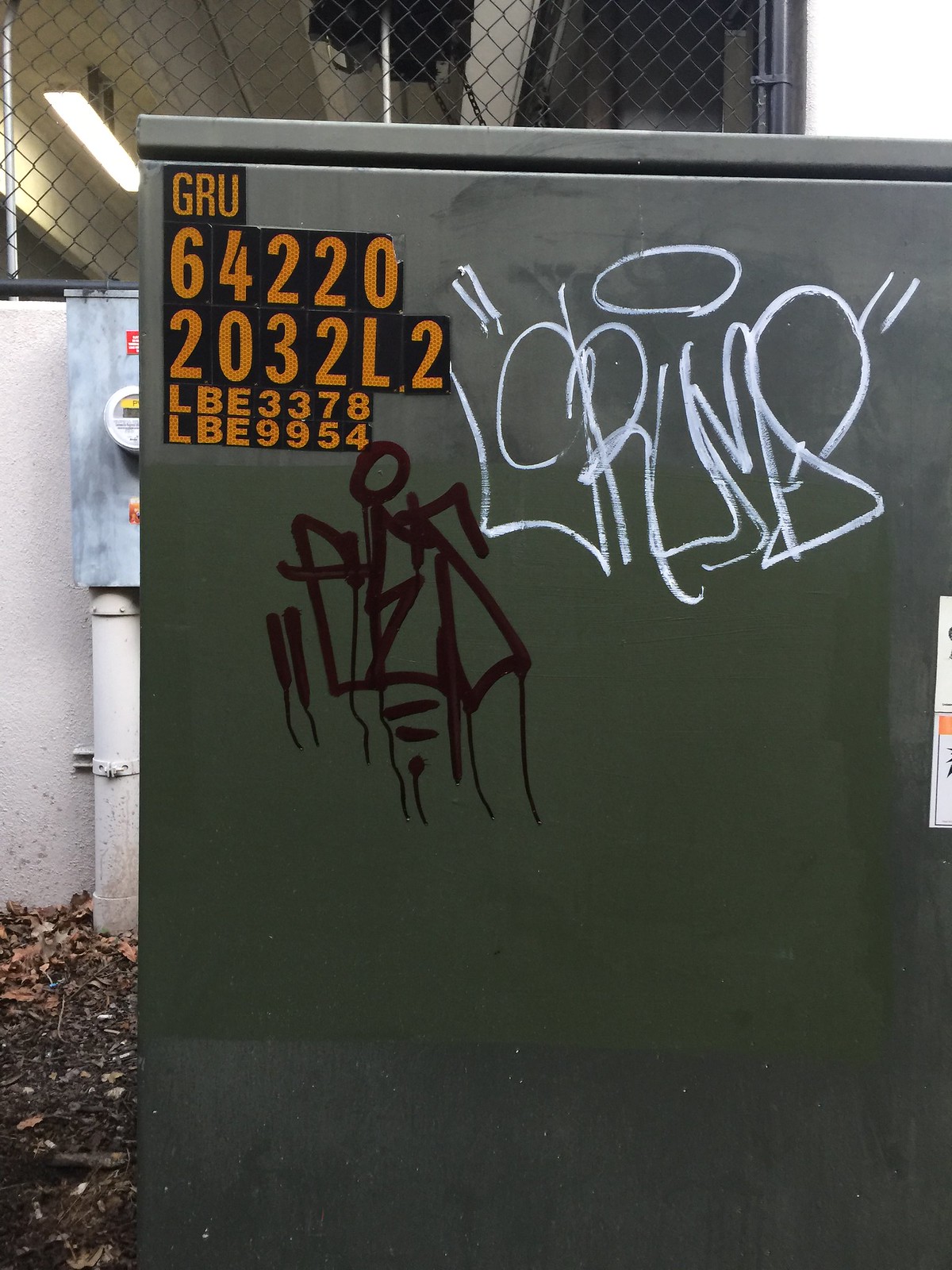The image is a vertically aligned rectangular photograph depicting the side of a dark green-gray utility box, which is likely used for providing electricity or other utilities. The majority of the photograph is dominated by this metal box, which features graffiti in both black and white paint, though the tags are not clearly readable. Notably, there is a white graffiti tag encased in quotation marks. In the upper left-hand corner of the utility box, there is a black sticker with orange text displaying the following details in bold print: “GRU,” followed by “64220,” “2032L2,” “LBE3378,” and “LBE9954.” 

The background offers a glimpse of the surrounding environment, featuring dirt and dried leaves in the lower-left corner. Above this, a stone wall painted white supports a chain-link fence. Adjacent to the utility box, there appears to be a meter, possibly a gas meter, situated in the middle of the frame. The overall scene suggests an outdoor setting, likely at the corner of a street or a similar location where such utility boxes are commonly found.